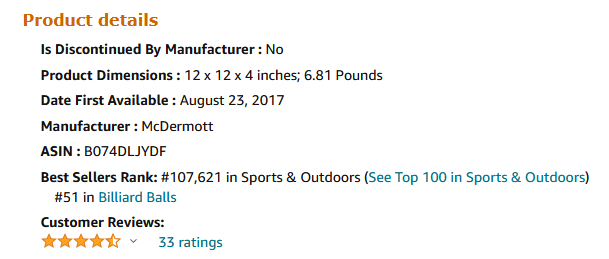A screenshot featuring a white background with product details highlighted in orange. The product has been discontinued by the manufacturer and lacks specified dimensions. Detailed information includes dimensions listed as 12 x 12 x 4 inches and a weight of 6.81 pounds. This item was available from MacDermott with an ASIN of B074DLJYDF and was first listed on August 23, 2017. It holds a Best Sellers Rank of 107,621 in Sports and Outdoors, with a top 100 position (#100) in the same category. Additionally, it is ranked #51 in the "Biller at the Bowls" category. The product has received an average customer rating of 4.5 stars from 33 reviews. All categorical and review-related information is depicted in blue text.